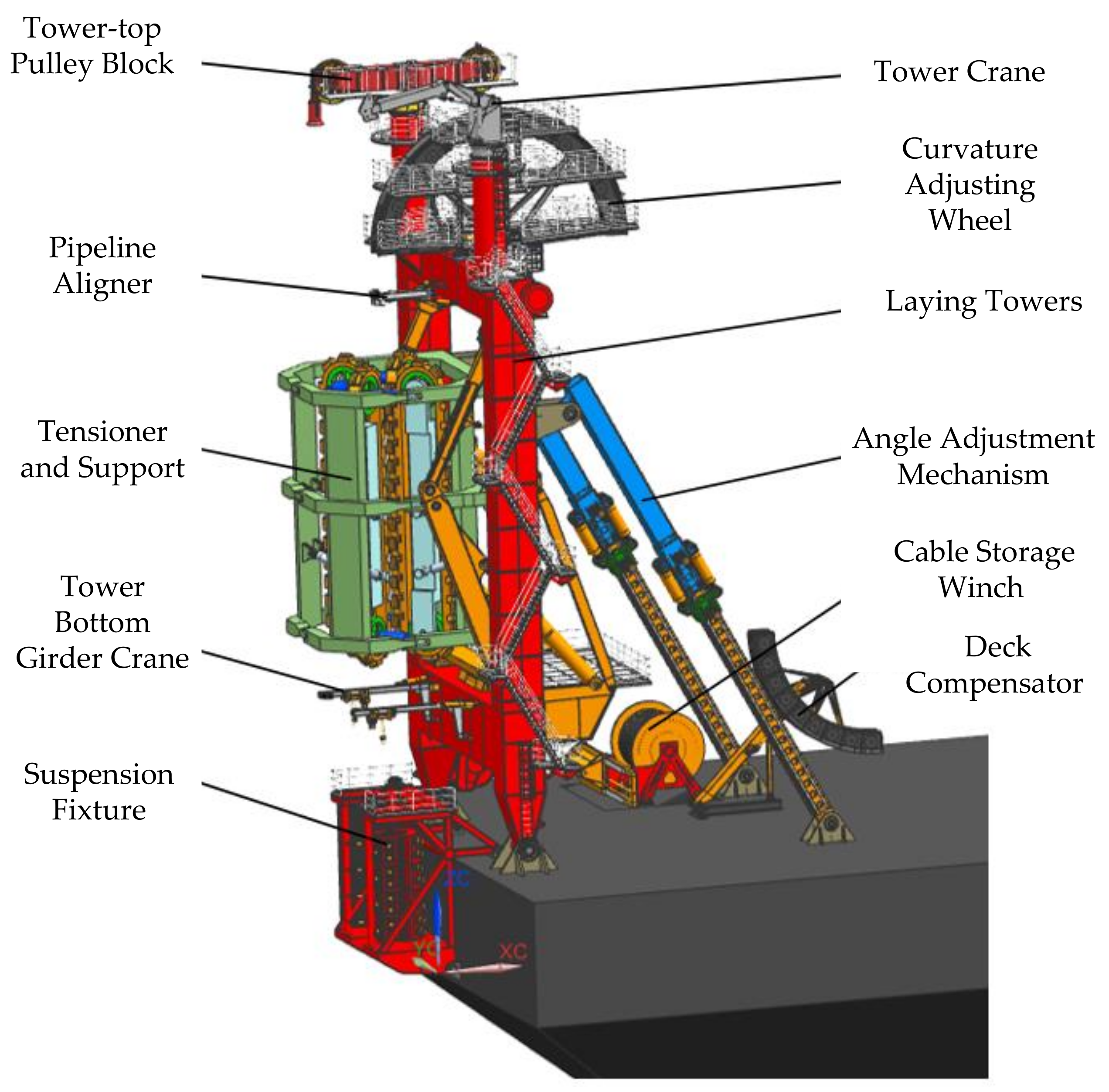The image is an intricate illustration of a large, industrial tower crane mechanism, prominently featuring various mechanical components in distinct, vibrant colors. The majority of the structure is painted fire engine red, with significant sections highlighted in construction equipment yellow, as well as parts in blue and green, all anchored to a solid, gray base. At the top of the crane is the "tower top pulley block," followed by the "pipeline aligner" directly beneath it. Lower down are the "tensioner and support," "tower crane," "curvature adjusting wheel," "laying towers," and "angle adjustment mechanism." Additionally, the machine includes a "cable storage winch" and a "deck compensator," with the "tower bottom girder crane" and "suspension fixture" completing the structure at the bottom. Each component is meticulously labeled, detailing its specific function and position. This massive, steel construction rises impressively high, showcasing the complexity and precision of its industrial engineering.